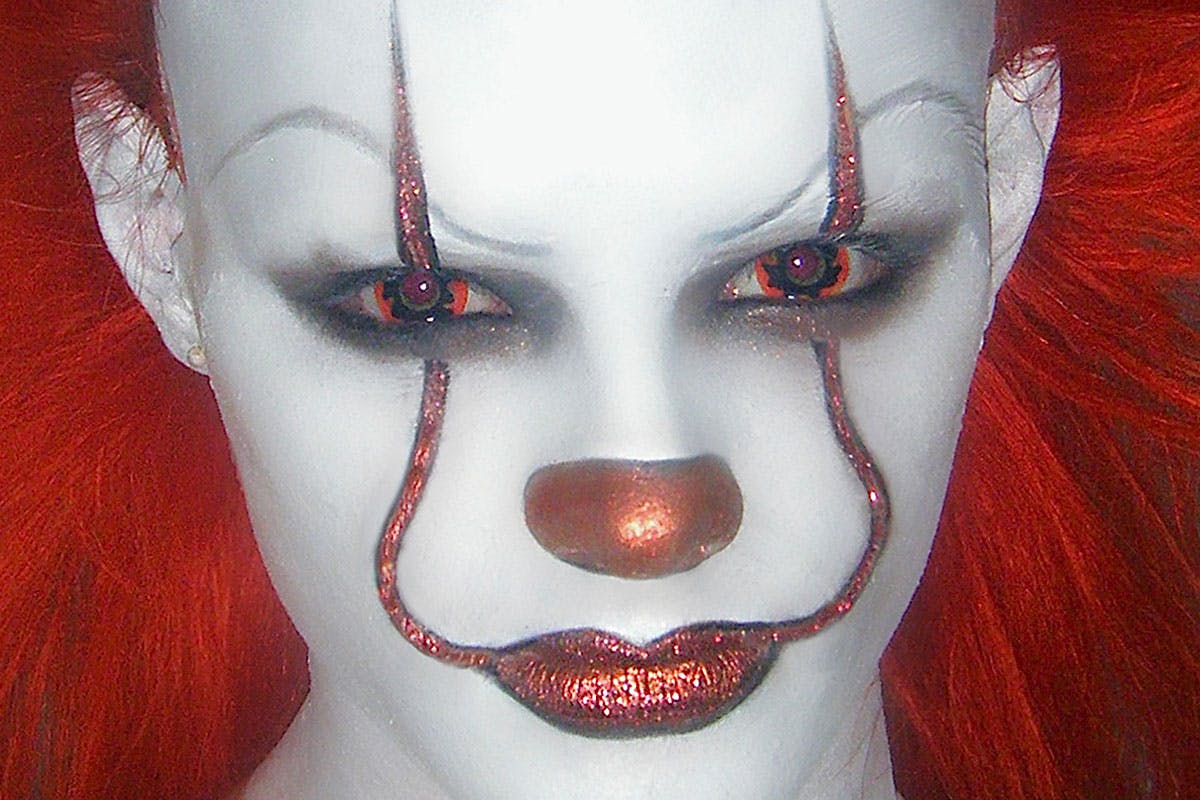The image is a close-up of a person with elaborate clown makeup, possibly female, featuring a bright red wig with straight hair that flares out from the face. The face is painted white, and the subject has high, arched eyebrows drawn prominently. The eyes feature striking contact lenses with red irises and black circles around the pupils. The tip of the nose is covered in red glittery paint, matching the shiny, almost glittery red lipstick that extends from the lips, curving up past the eyes and becoming pointier beyond them. There is dark gray makeup around the eyes, adding to the intense look. The overall style resembles a character from "It," giving the clown an eerie and potentially sinister appearance. The makeup and the vivid colors make it unclear whether this is a real photograph, a 3D image, or even a foam mannequin.